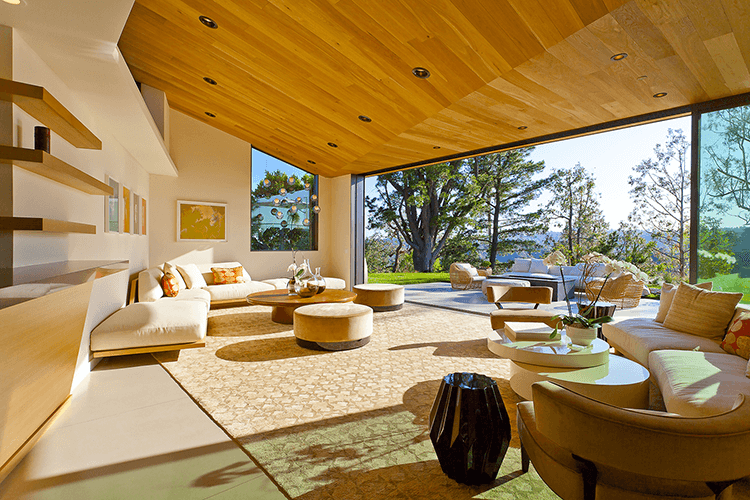This photograph looks straight out of Architectural Digest, capturing the essence of a luxurious modernist home interior. The room features wood-paneled ceilings with intricate angles and recessed lighting, complemented by an impossibly large, floor-to-ceiling glass wall that bathes the space in natural sunlight. The white-painted walls are adorned with a few pictures, specifically on the far left wall where four colorful images hang: one blue, two orange, and one brown. Another picture depicting green leaves is placed on an angled wall. 

The interior presents a sophisticated, minimalistic decor, showcasing an assortment of modern furniture, including low round ottomans, low chairs with curved backs, a round coffee table, and uniquely shaped oval coffee tables. The seating arrangement is anchored by an expansive cream and tan patterned area rug. Some sofas are built into the wall with matching free-standing sofa pieces, all covered with white cushions and accented with red and gold pillows. 

There are floating bookshelves with minimal adornments situated behind one of the built-in sofas. Additionally, there's a striking white, eight-shaped coffee table holding a book and a plant. A dark black vase adds a touch of elegance, and round tan cushions lie next to the coffee table. 

The room opens up to an outdoor deck through the massive glass wall, revealing a concrete patio set amidst a grassy lawn and lush trees – a private, serene landscape. The patio is furnished with a large white sofa, tan wicker chairs with cushions, and a central table or possibly a barbecue grill. In the far background, the view extends to the ocean, further emphasizing the exclusivity and aspirational quality of this stunning modern house.